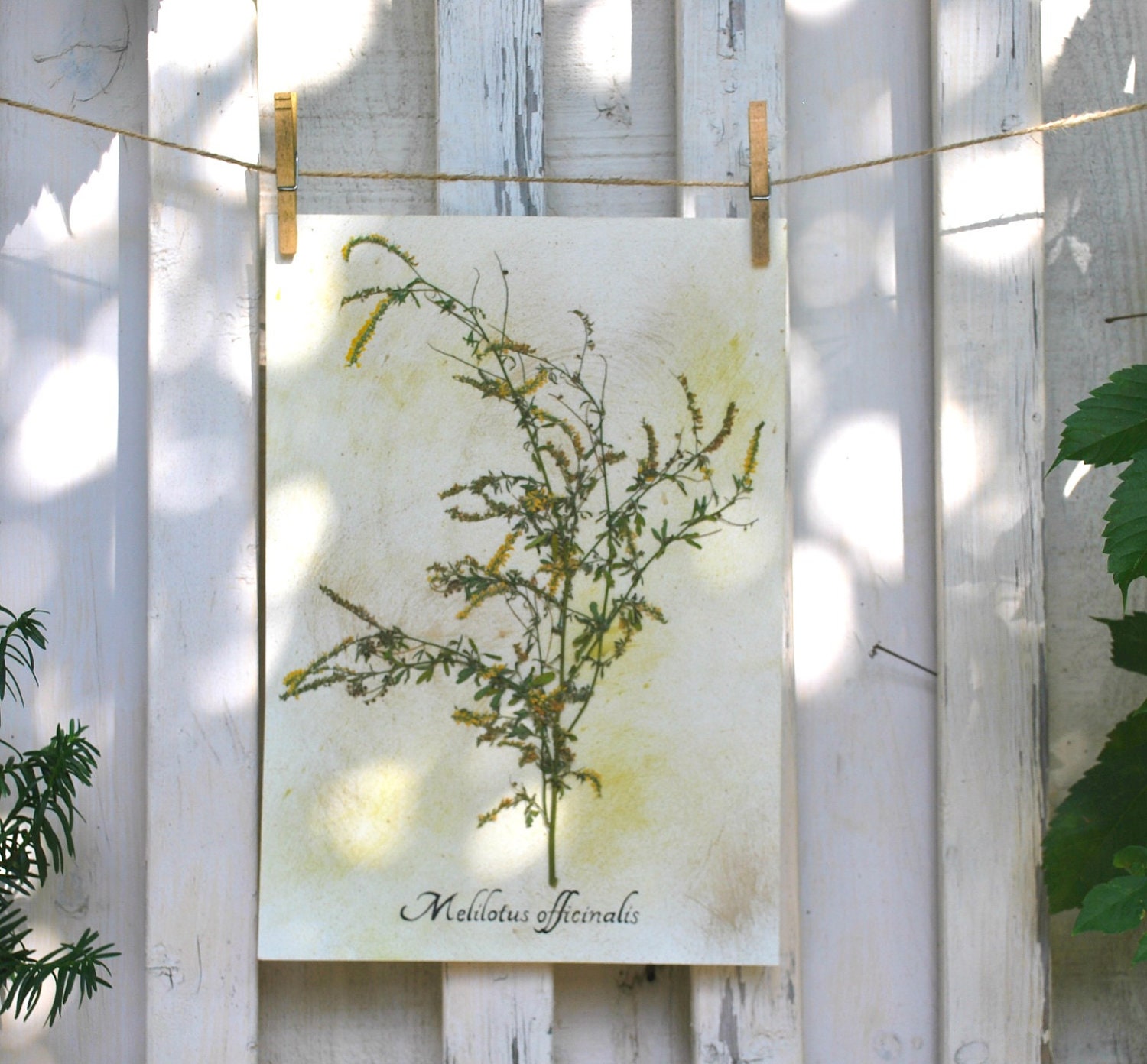This is a photograph depicting a detailed botanical artwork hanging outdoors against a white painted fence. The artwork, labeled "Melilotus officinalis" in black curvy text at the bottom, is mounted on a white canvas and suspended by a piece of thin, simple rope that stretches across the top of the image. The rope, with a slight dip in the center, is fastened with two beige wooden clothespins featuring silvery clasps. The painting itself showcases a plant with slender green stems that angle slightly to the left, branching off at 45-degree angles and adorned with narrow green leaves and clusters of tiny, elongated yellow flowers. Surrounding the canvas, the photograph captures the lush greenery of actual plants, with larger green shrubbery to the right and a smaller plant with narrow leaves to the left. The scene is bathed in soft, dappled sunlight, enhancing the overall tranquil and natural ambiance.